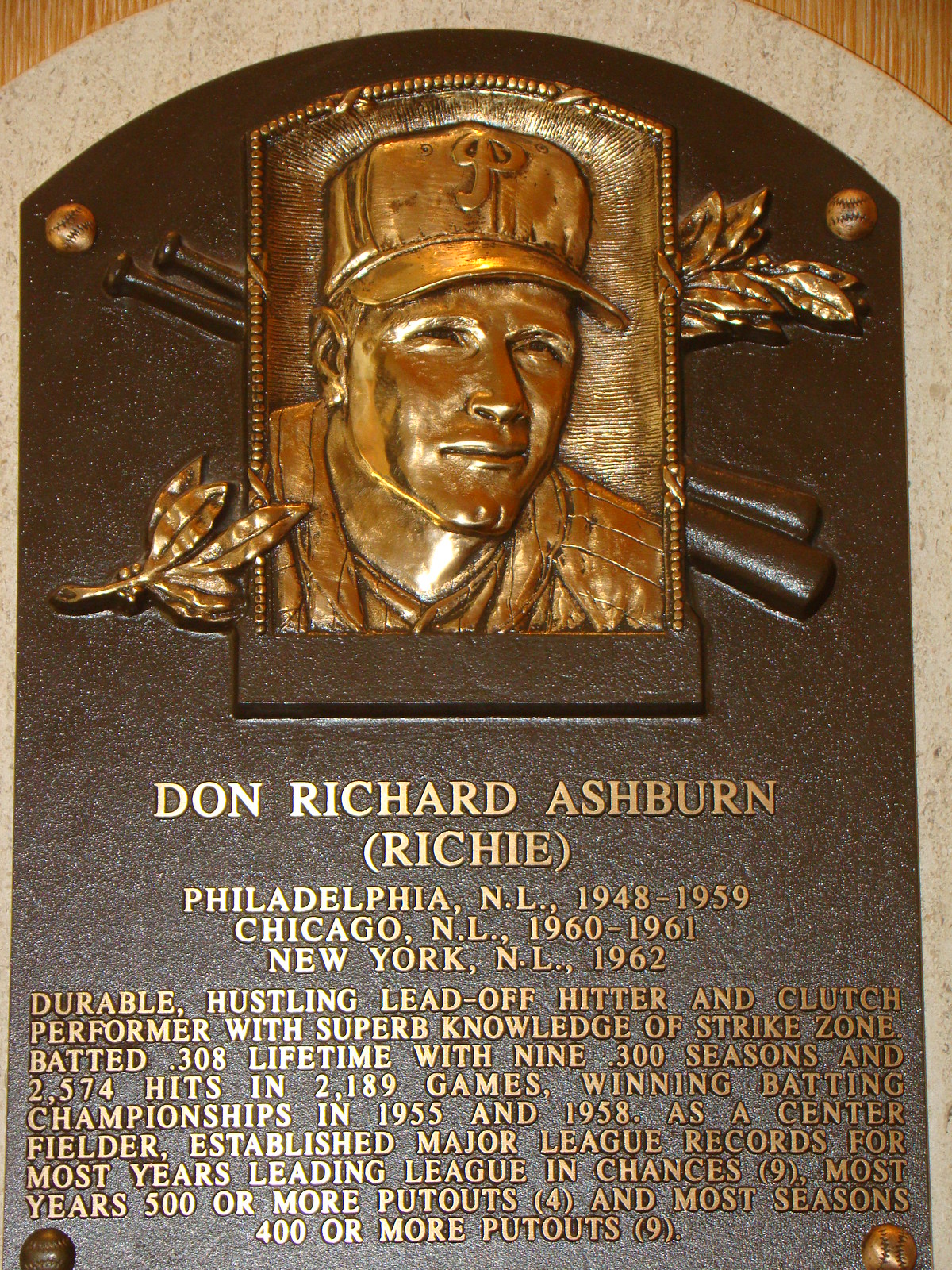The image features a detailed bronze and brown plaque, prominently displayed against a wooden background, likely in an indoor museum setting. At the center of the plaque is a bronze relief depicting a male baseball player wearing a cap with a 'P' on it, signifying the Philadelphia Phillies. Behind the player's face are two crossed baseball bats, with bronze baseballs serving as rivets in each of the four corners of the plaque.

The plaque honors Don Richard Ashburn, also known as Richie, who played for three major teams: Philadelphia National League from 1948 to 1959, Chicago National League from 1960 to 1961, and New York National League in 1962. It highlights his impressive career as a durable, hustling leadoff hitter with a superb knowledge of the strike zone. His remarkable statistics include a .308 lifetime batting average, nine seasons with over .300 batting averages, and a total of 2,574 hits in 2,189 games. The text goes on to note his accomplishments in batting championships, having won in 1955 and 1958, and setting major league records as a center fielder for the most years leading the league in chances (nine), most years with 500 or more putouts (four), and most seasons with 400 or more putouts (nine).

The plaque’s colors include shades of brown, off-white, dark brown, gold, and bronze, enhancing its detailed and commemorative nature. The object dominates the entirety of the photographic frame, making its historic and artistic details clearly visible.